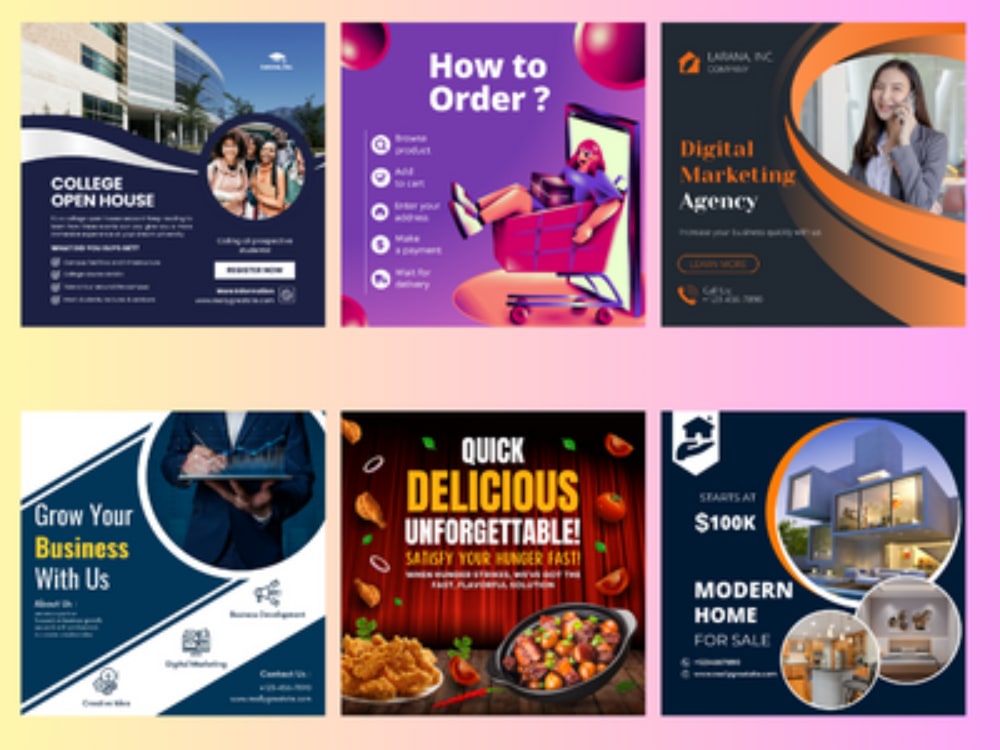The image is an innovative graphic design advertisement featuring six distinct promotional designs, arranged in a grid of three rows and two columns, against a vibrant background that transitions from yellow on the left to pink on the right with a faded gradient effect. Each design is showcased within a square, offering a diverse range of advertising concepts:

1. **College Open House**: Located at the top left with a navy blue theme, this advertisement includes images of people and buildings inside a circular frame, alongside text with bullet points and a couple of lines introducing the event.
   
2. **How to Order**: Positioned at the top center, this ad has a purple background with a whimsical cartoon style, depicting a person sitting in a shopping cart and offering instructions on ordering processes.
   
3. **Digital Marketing Agency**: The top right square presents this ad against a black background, featuring a professionally dressed woman on a phone call, suggesting business-oriented services.
   
4. **Grow Your Business with Us**: Situated at the bottom left, this advertisement focuses on business growth and features a headless figure writing on a clipboard.
   
5. **Quick Delicious Unforgettable**: Centered on the bottom row, this culinary-themed ad with a dynamic depiction of food in a pan highlights quick and delicious menu options, aimed at satisfying hunger promptly.
   
6. **Modern Home for Sale**: The bottom right ad advertises homes starting at $100,000, displaying the exterior and interior views of a modern house within circular frames.

The entire arrangement suggests a digital or magazine format, providing a comprehensive visualization of various advertisement styles for potential selection.